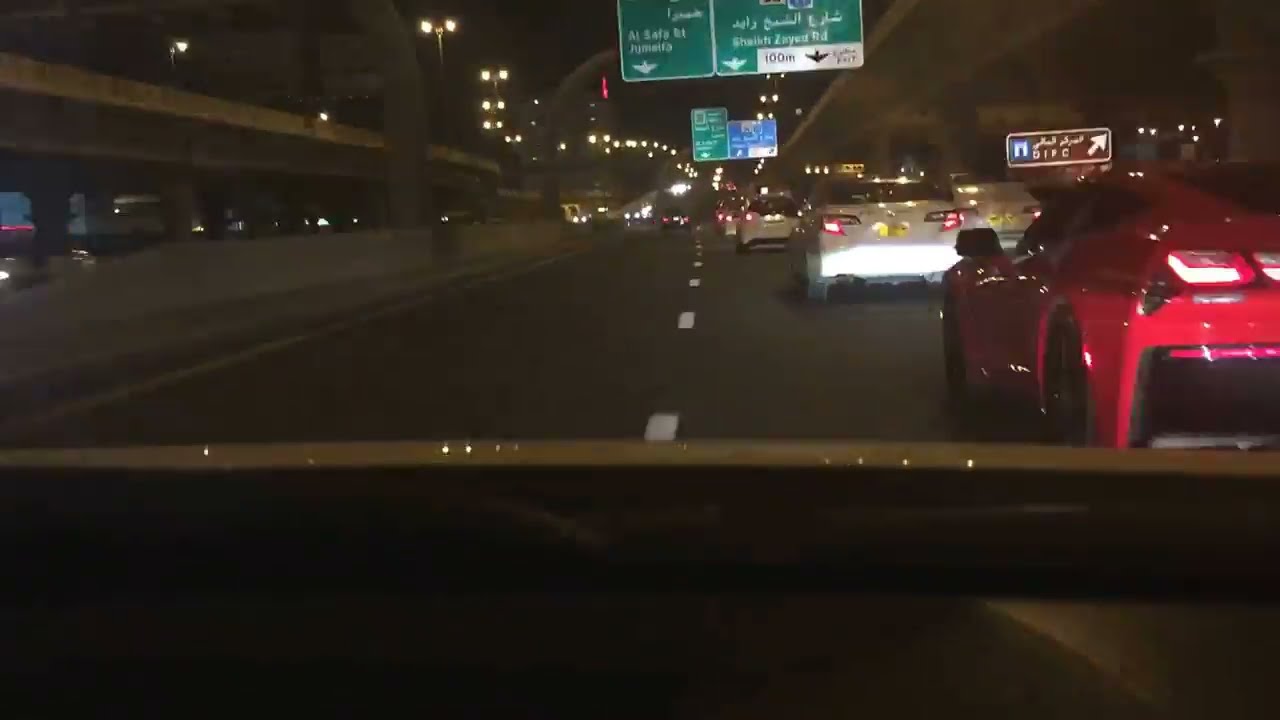The photograph captures a bustling nighttime freeway scene from inside a vehicle, with the dashboard visible in the immediate foreground. The road is populated with numerous cars, predominantly white, with one prominent red sports car directly ahead. Streetlights illuminate the scene, casting a white glow over the vehicles. Overhead, green street signs display white text, including directional arrows and distances in meters, indicating upcoming exits. A brown sign on the right hints at a point of interest. The highway is marked with white lane dividers, guiding the flow of traffic. Yellow license plates on the cars suggest a non-U.S. location, and the dark night sky forms a stark backdrop. The driver appears to be maneuvering from the left lane toward the right, navigating through this well-lit, well-marked urban expanse.